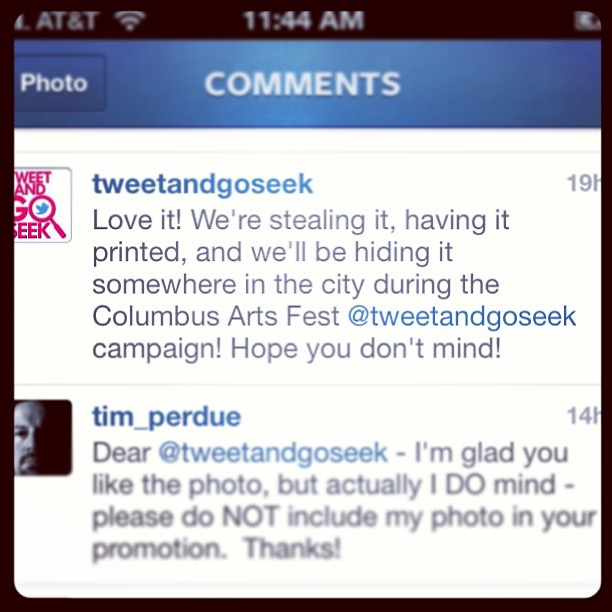This is a detailed screenshot taken on a phone, displaying a Twitter interaction. At the top left corner, it shows the AT&T network with three bars of service, a time stamp of 11:44 AM in the center, and a partially visible battery indicator on the right side. The upper section has a black border around the entire image, and immediately below, there's a blue bar that features the words "Photo" and "Comments" in white.

The central content of the screenshot is comprised of two tweets set against a white background. The first tweet is from "Tweets and Go Seek," which reads: "Love it, we're stealing it, having it printed, and we'll be hiding it somewhere in the city during the Columbus Arts Fest at Tweets and Go Seek campaign. Hope you don't mind." This tweet was posted 19 hours ago.

Beneath this tweet is a response from Tim Perdue, which features a small profile picture of a man. Tim Perdue's tweet states: "Dear @Tweets and Go Seek, I'm glad you like the photo, but actually, I do mind. Please do not include my photo in your promotion. Thanks." This tweet was posted 14 hours ago. The content highlights a disagreement where Tim Perdue requests that his photo not be used by Tweets and Go Seek for promotional purposes during the Columbus Arts Fest.